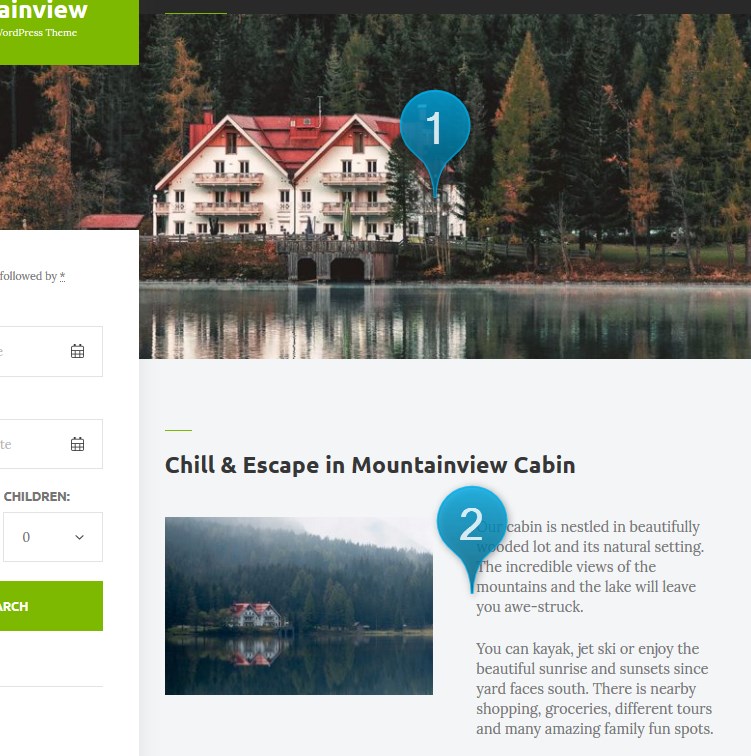**Image Description:**

The image appears to be a screenshot from a website, possibly a real estate or vacation rental site. The layout is divided into several sections:

- **Top Left Corner:** There's a partial view of a green box with the text "AimView" partially visible along with some smaller, unreadable writing. This could potentially be a website feature or branding element related to platforms like WordPress or Twitter.

- **Main Section:** Dominated by a large photograph of a picturesque house. The house features a distinctive red roof and two balconies, set against the backdrop of lush woodland. In front of the house, there is a body of water, possibly a river, and a bridge extending to the right.

- **Calendar and Booking Box:** Below the main image or within the same section is a white box, likely containing calendar icons indicative of booking availability. This section probably allows users to make reservations.

- **Button:** A green button is visible at the bottom of the booking box, which likely serves as the call-to-action for booking or inquiring further.

- **Location Markers and Description:** To the right of the main image, there's a blue marker with the number "1" in white, resembling a location pin. Below this marker, there's a tagline on a white background: "Chill and escape in Mountain View cabin." Another blue marker with the number "2" appears, paired with an extensive description of the cabin.

**Description of the Cabin:**
- "Situated in a beautifully wooded lot with incredible mountain and lake views, this cabin offers awe-inspiring scenery. Guests can enjoy various activities like kayaking and jet skiing, along with stunning sunrises and sunsets thanks to the yard's southern exposure. Nearby, you can find shopping centers, grocery stores, diverse tours, and numerous family-friendly attractions."